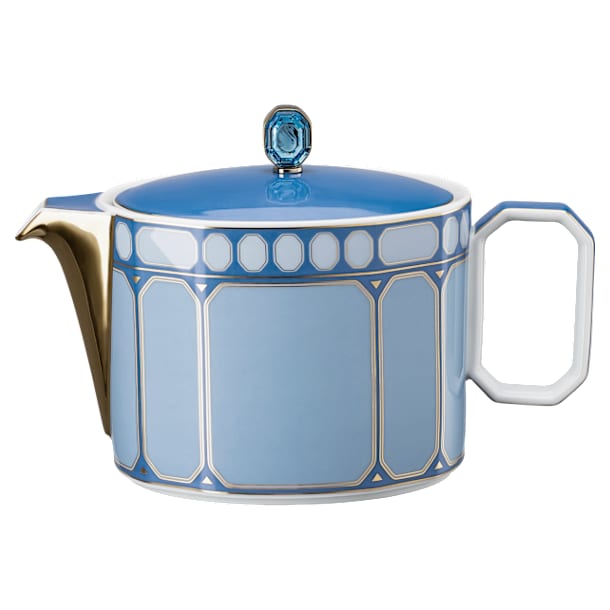This image displays a highly detailed, decorative teapot on a white background, seemingly designed more for display than practical use. The teapot itself is predominantly blue with an intricate array of geometric designs, including circles, vertical stripes, ovals, squares, rectangles, and even octagon shapes, all in varying shades of blue and silver. The spout is a shiny metallic silver with a hint of blue on its top, resembling a short, nostril-like nose and is positioned to the left. The teapot's handle is white on the inside and blue on the outside, shaped somewhat like a rectangular octagon. The lid of the teapot is dark blue and features a small, blue gemstone-like piece, likely glass, attached with a silver base. The overall condition of the teapot seems pristine, with no apparent damage, indicating it's likely an ornamental piece rather than one for everyday use.